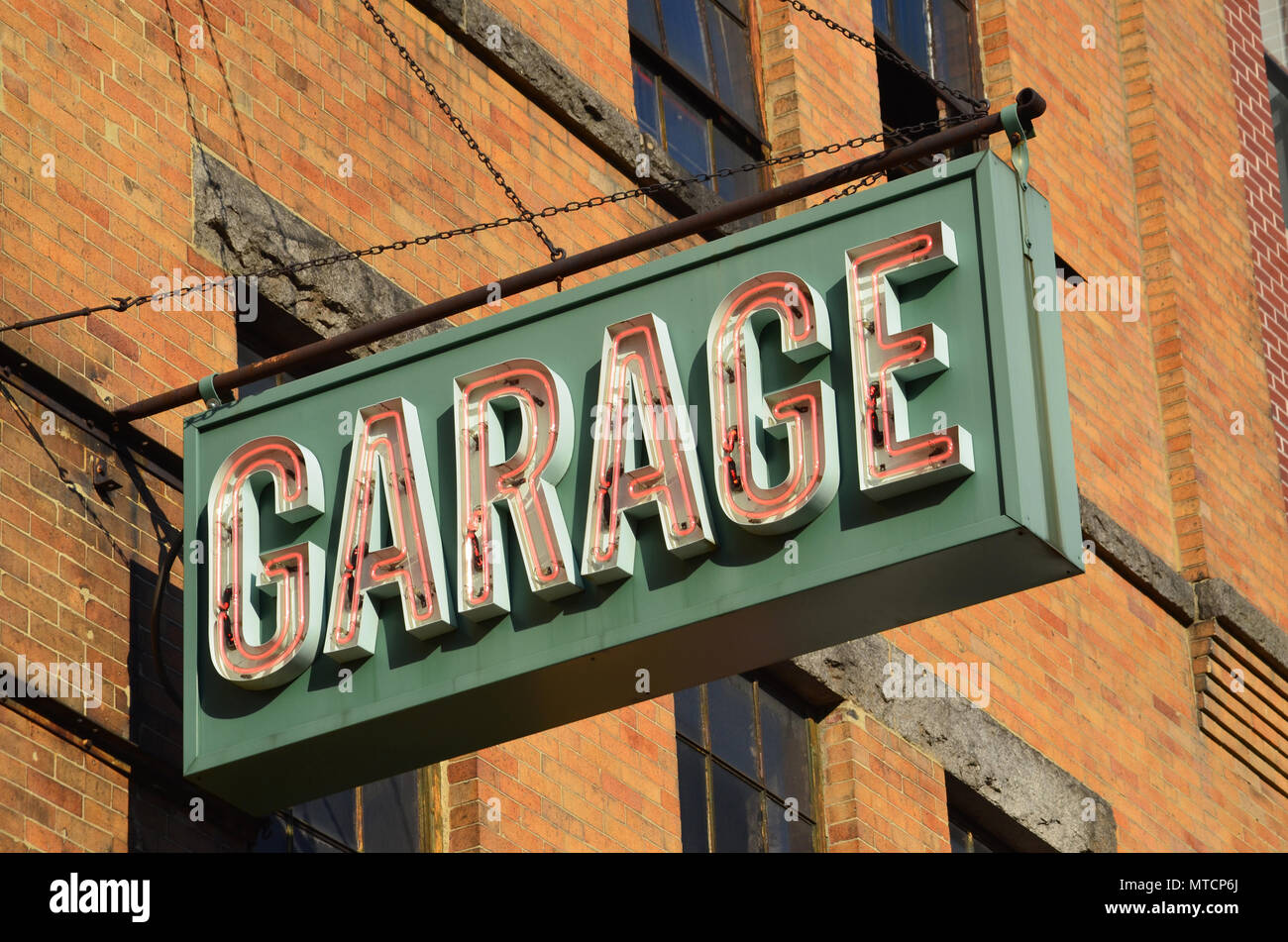This photograph captures a detailed image of a rusted metal rod extending horizontally from an orange brick building at a shallow angle to the frame. The rod supports a heavy, rectangular sign in sand green—often mistaken for sage green—hanging down by two matching hooks and additional stabilizing chains. The sign's border and background share the same sand green hue. Red neon lights housed in metal boxes spell out "GARAGE" across the sign in tall, narrowly spaced capital letters, making for a striking visual contrast. The brick building itself shows its age, with older cement cappings visible above several industrial-style windows, reinforcing the structure. The entire image is covered with a prominent, repetitive watermark that reads "Alamy" in transparent white text, alongside numerous scattered lowercase "a"s. Additionally, a black bar running along the bottom edge contains white text: "Alamy" on the left, "Image ID MTCP6J" and "www.alamy.com" in slightly thicker font on the right. The perspective suggests that the photographer looked up at a steep angle, indicating the sign is positioned roughly 10 to 12 feet above the ground.